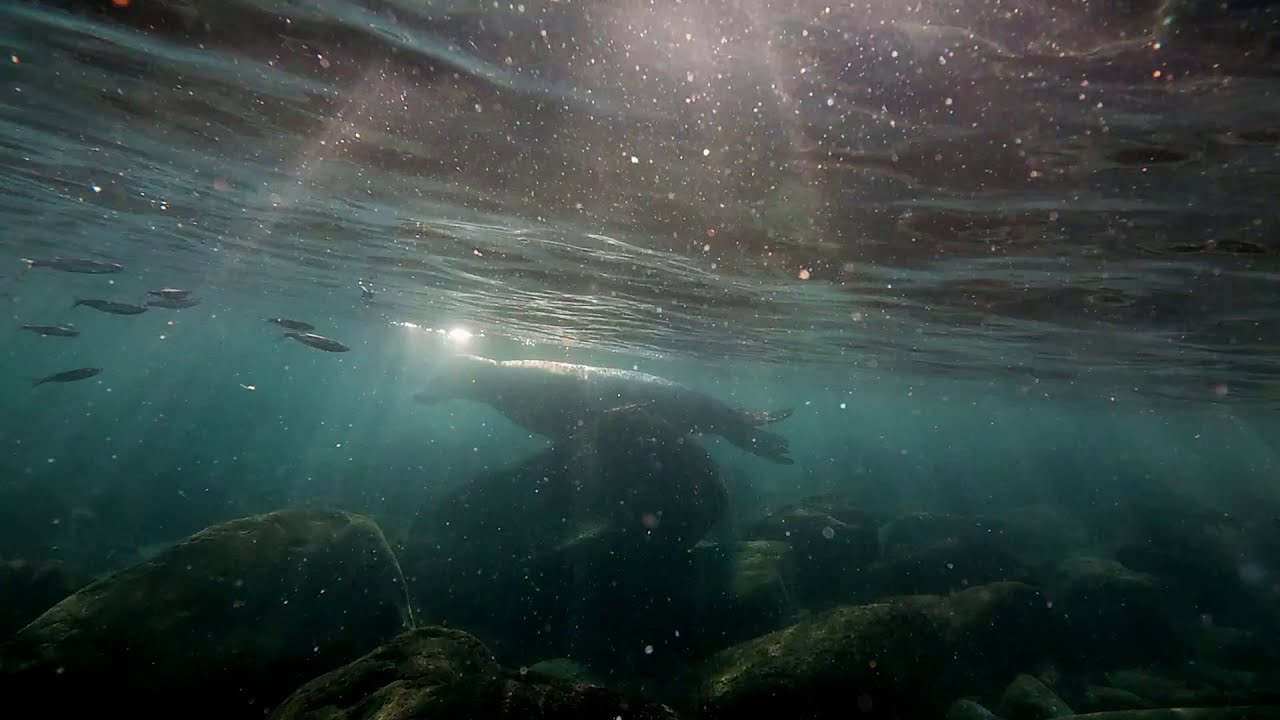Underwater, beams of sunlight pierce through the turquoise-tinted water, creating a mesmerizing play of light that illuminates the scene. The focal point of the image is a seal, swimming with its head towards the left side of the frame, its sleek form gliding gracefully in the center. Surrounding it, a school of eight to nine fish swim in the opposite direction, their silvery bodies reflecting the sunlight as they head towards the right. The scene is set against a backdrop of large boulder rocks at the bottom, covered in green algae and other growths, hinting that this is likely a shallow coastal area. Small particulates float through the water, catching the light and adding a dynamic texture to the scene. The upper part of the image is darker, with a mix of deep blue and dark hues, interspersed with wavy patterns indicating the surface above. The entire tableau suggests a late evening, adding a touch of mystery and tranquility to this underwater snapshot.